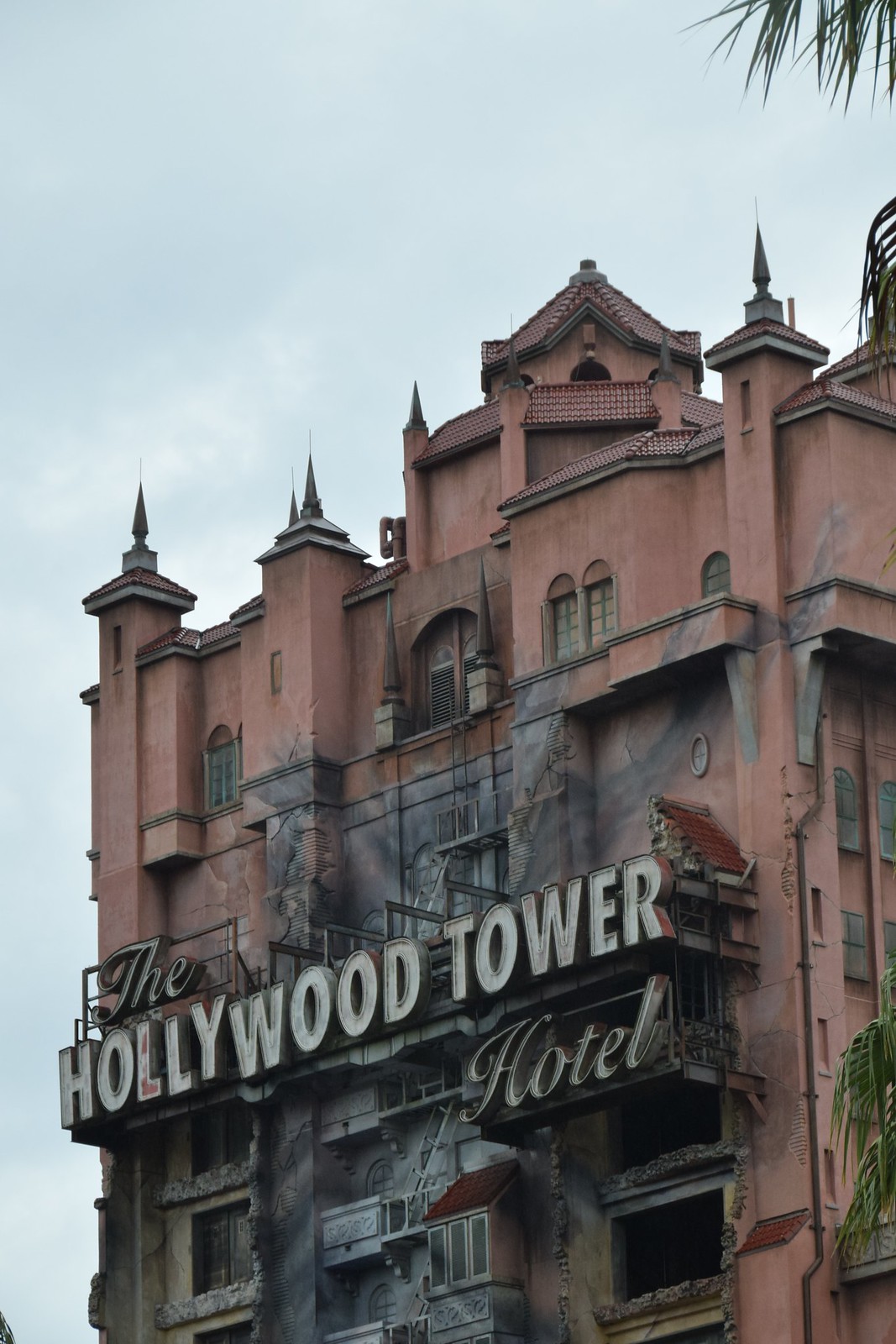The image depicts the Hollywood Tower Hotel located at Disney World's Hollywood Studios in Florida. Dominating the bottom right corner of the portrait-oriented photograph, the building's exterior is predominantly a burnt, reddish-brown color, accented by areas of scorched black, possibly from a fire. The centerpiece of the facade is a neon sign bearing the cursive word "The" followed by the bold, capitalized words "Hollywood Tower," with "Hotel" written underneath. Steeples and what may be lightning rods adorn the roof, contributing to the building's turn-of-the-century architectural feel. The sky in the upper left portion of the photo is bluish and slightly hazy, providing a stark contrast to the hotel's eerie, aged appearance. In the upper right corner, a hint of palm fronds peeks into the frame, while greenery suggests a treetop at the building's right edge.